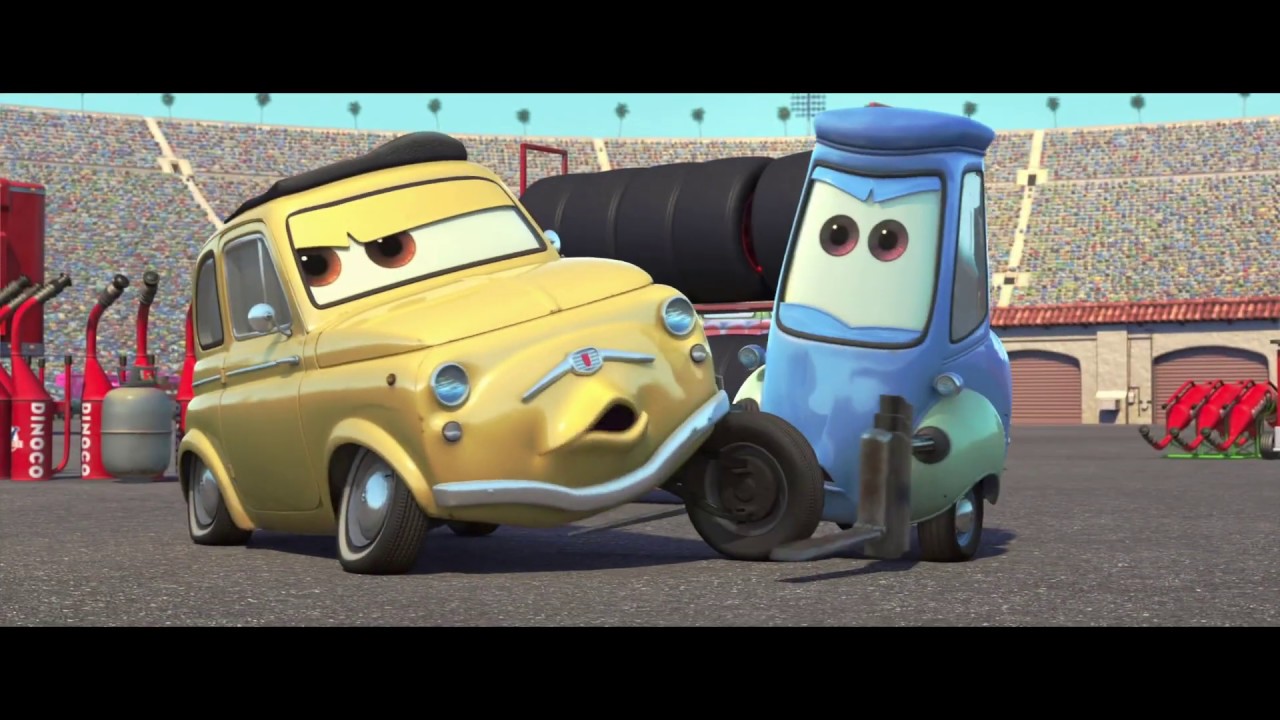This is a detailed scene from the Pixar Disney movie *Cars*, where the vehicles are anthropomorphized with eyes on the windshields, grills that resemble mouths, and expressive wheels. In this cinematic clip, framed by thick black borders at the top and bottom, the focus is on a pit stop setting. The central characters are two Italian cars: Guido, a small blue forklift, and Luigi, a vintage yellow car featuring chrome hubcaps, chrome bumper, small round headlights, and stylish white-walled tires.

In this specific frame, Guido is in the process of changing Luigi's tire next to a rack of race tires, emphasizing a teamwork dynamic reminiscent of a real pit stop. The background reveals a bustling stadium filled with spectators, exuding the energy of a major race event. Closed garage doors and numerous red and gray fuel cells labeled "DIN-O-CO" in white add further authenticity to the racing environment. This scene captures the vibrant and dynamic world of *Cars*, blending lively character interactions with detailed automotive elements.